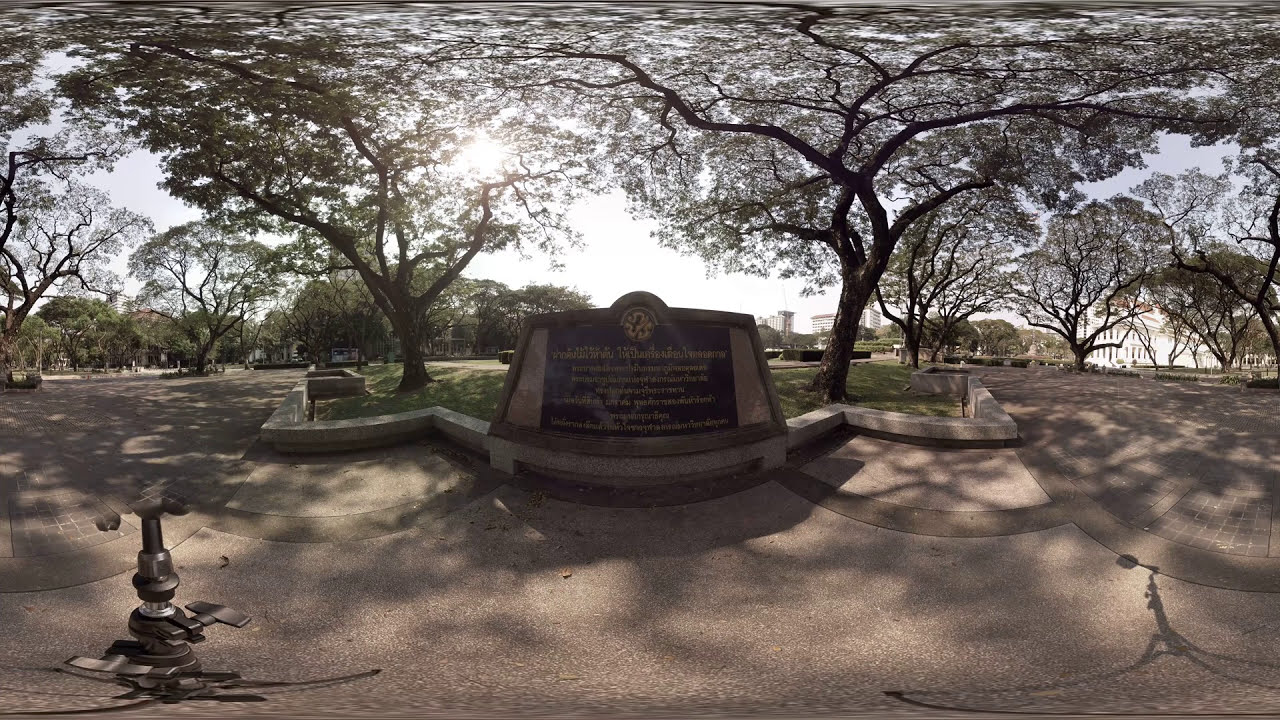The image captures a 360-degree panoramic view of an outdoor memorial or tomb situated in what appears to be a central park in an urban environment. The large, black stone structure stands prominently in the center with inscribed writings in a non-English language, featuring a hint of gold or bronze. At the top of the monument is a distinctive medallion. Flanking the memorial are two trees with lush green leaves, suggesting a summer or pleasant weather setting, under a clear, blue sky with no clouds. In the background, skyscrapers rise far in the distance, indicating the park's urban locale. The foreground reveals a decorative paved walkway, with sections of concrete and paver bricks, some of which show signs of cracking. Additional observed details include the camera's support stand at the bottom left, casting a shadow in the bottom right corner of the image. There are no people present, highlighting the monument's serene and solemn atmosphere.